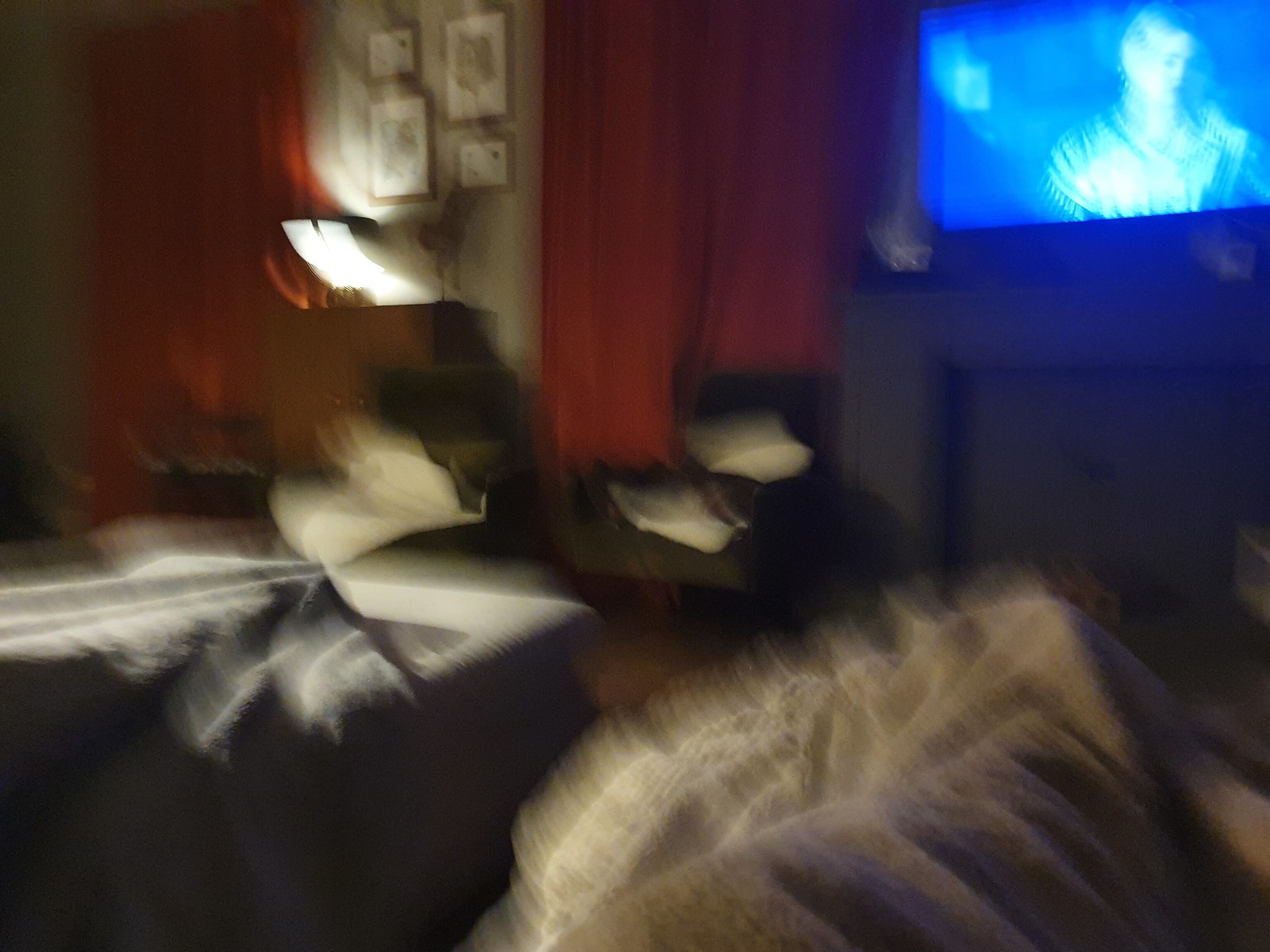This image captures a cozy living room scene. The space features a grey couch and multiple chairs, which appear to be in shades of green, though the lighting makes the exact color difficult to determine. A television is on, displaying a character against a bright blue background. The room is decorated with red and orange drapes and several small paintings on the wall. On the carpeted floor, there are blankets, adding a homely touch. A nightstand or cabinet is situated nearby with a lamp perched on top, illuminating the room gently. Overall, the environment exudes the warmth and comfort of a lived-in space.